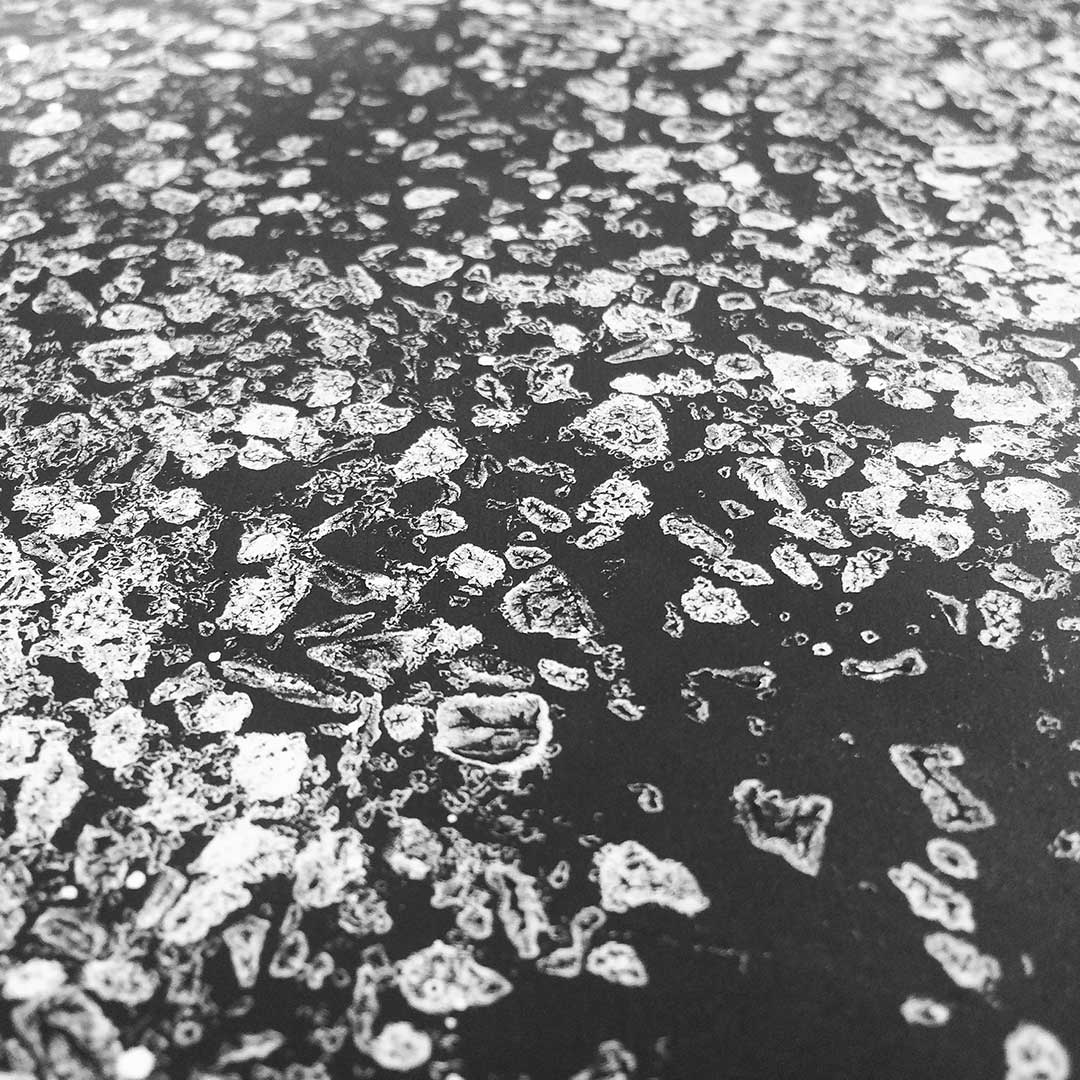The image appears to be a black and white microscopic view of a densely packed slide, likely showcasing numerous tiny microorganisms or potentially crystalline structures scattered across it. The background is dark, creating a stark contrast with the chalky white, circular, and splotchy objects that dominate the scene. These small, fingerprint-sized entities are distributed throughout the image, with a noted concentration in the upper right section, tapering off towards the lower right, which appears a bit more open. The upper left-hand corner is slightly blurry, adding to the chaotic yet structured aesthetic of the microscopic view. The overall scene resembles a crowded landscape of cultured microorganisms or crystalline formations, floating and seemingly attempting to move within their confined space.